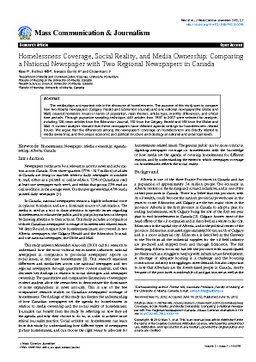**Screenshot of a Document Titled 'Mass Communications and Journalism'**

This detailed screenshot captures a document that appears to be either a photo or a screenshot of a text. The document is titled "Mass Communications and Journalism," with the title positioned in the top left corner. Directly beneath the title, there is a black bar spanning the width of the document, providing a visual break.

In the same top left area, additional information is provided, including the address and email of the associated companies.

The focal content of the document is an article or open letter titled "Homelessness Coverage: Social Reality and Media Censure." This article apparently examines how homelessness is portrayed by the media, specifically including perspectives from a national newspaper and two regional newspapers in Canada. The author's information is displayed prominently as well.

Below the main title, there is a boxed section labeled "Abstract," which serves as a concise summary, similar to a "too long; didn't read" (TL;DR) overview of the article.

The body of the document consists of five well-structured paragraphs, likely elaborating on the topic, providing insights, analysis, and possibly data.

At the bottom right corner, source information is provided, complete with hyperlinked references, suggesting this might be part of a website entry. The presence of hyperlinks allows readers to easily access the cited sources for further reading or verification.